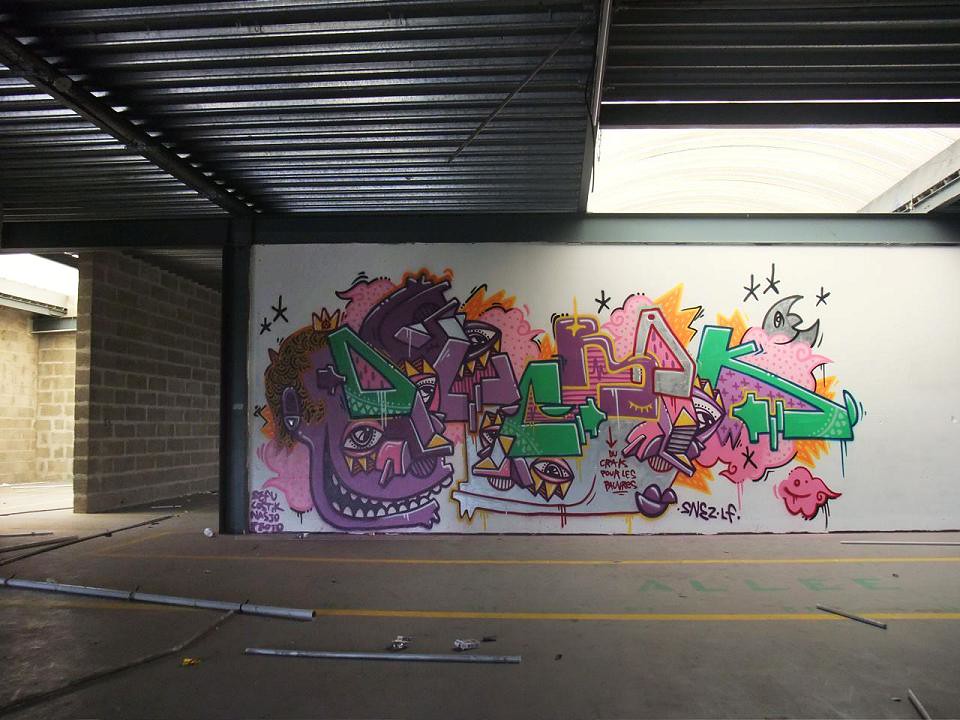The image depicts an underground parking garage featuring a white wall adorned with vivid graffiti. The scene is framed by structural metal beams and a red brick wall extending from the left toward the center. The concrete floor, marked by two yellow lines running through the middle, adds to the urban decay vibe, and various metal rods and tubing are scattered on the ground.

The graffiti itself is a striking array of colors, predominantly featuring pink, purple, green, with splashes of light orange, gray, and brown. On the far left of the wall, there's a distorted yet distinguishable figure outlined in purple, possibly representing a person with two eyes. Nearby, text resembling "DCK" or possibly "D-C-R-O-K" is scrawled, with the letters in green, purple, and gray.

In the center of the wall, a peculiar purple face stands out, which some observers liken to a disfigured human form or even a smiling monkey with yellowish hair. Alongside this, another similar face appears, both encircled by vivid pink accents. Towards the right, the graffiti explores more abstract themes, featuring a crescent moon with a hole, pink clouds, various green triangles, and some nearly illegible text. The entire piece blends chaotic color with urban grit, creating an arresting visual experience.